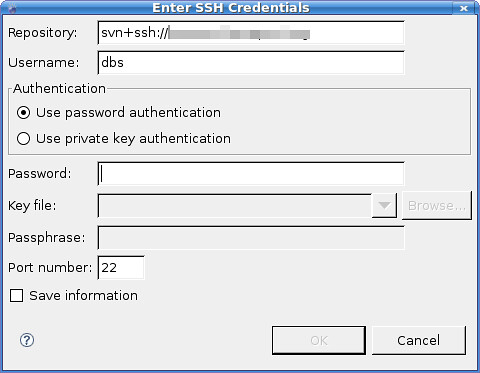The image depicts a screenshot from a computer screen, showing a pop-up window for entering SSH credentials. The window, characterized by a blue border and a blue header that reads "Enter SSH credentials," features an 'X' logo in the top-right corner, allowing the user to close it. Below the header, there are several fields enclosed in white rectangles for user input. The first field asks for the "Repository," which is noted to be formatted as "svn+ssh://". Beneath this, there are input fields labeled "Username" and a section for "Authentication." Users can select either "Use Password Authentication" or "Use Private Key Authentication," with the example showing "Use Password Authentication" selected. Following the authentication method, there are spaces to enter a "Password," although some greyed-out boxes indicate areas where text cannot be entered. Additional fields request a "Key File," a "Passphrase," and a "Port Number," which defaults to "22." At the bottom of the window, there are options for "Save Information" and buttons to either "Enter" or "Cancel" the process. Notably, there are several blank spaces throughout the form, indicating incomplete inputs.